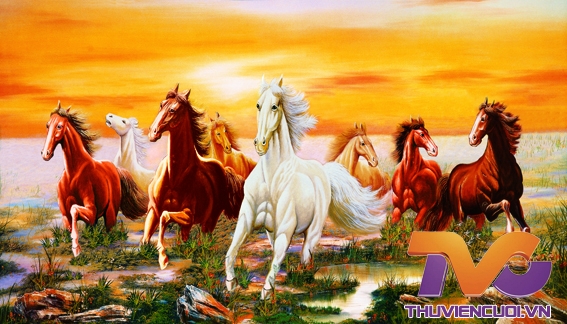This vivid color image likely from a Vietnamese network, identifiable by the watermark "tvc, thuviencoi.vn" in the bottom right, showcases a picturesque scene at sunset featuring a bunch of eight wild, cartoonishly drawn horses. The sky is a striking blend of orange and yellow, with accents of reddish-brown and hints of a setting sun. The background includes what appears to be a reflective body of water, tinged with light pink tones under the glowing sky. 

The foreground of the image consists of patches of green grass interspersed with small pond-like bodies of water. The horses are spread across this area, each depicted with a muscular build and flowing manes and tails. The central horse is distinctly white, flanked by various shades of brown tan, and two additional white horses positioned slightly behind. Each horse appears to be in mid-motion, capturing a dynamic moment as if caught in the midst of running. The artistic detail vividly brings to life the strength and majesty of these wild creatures.